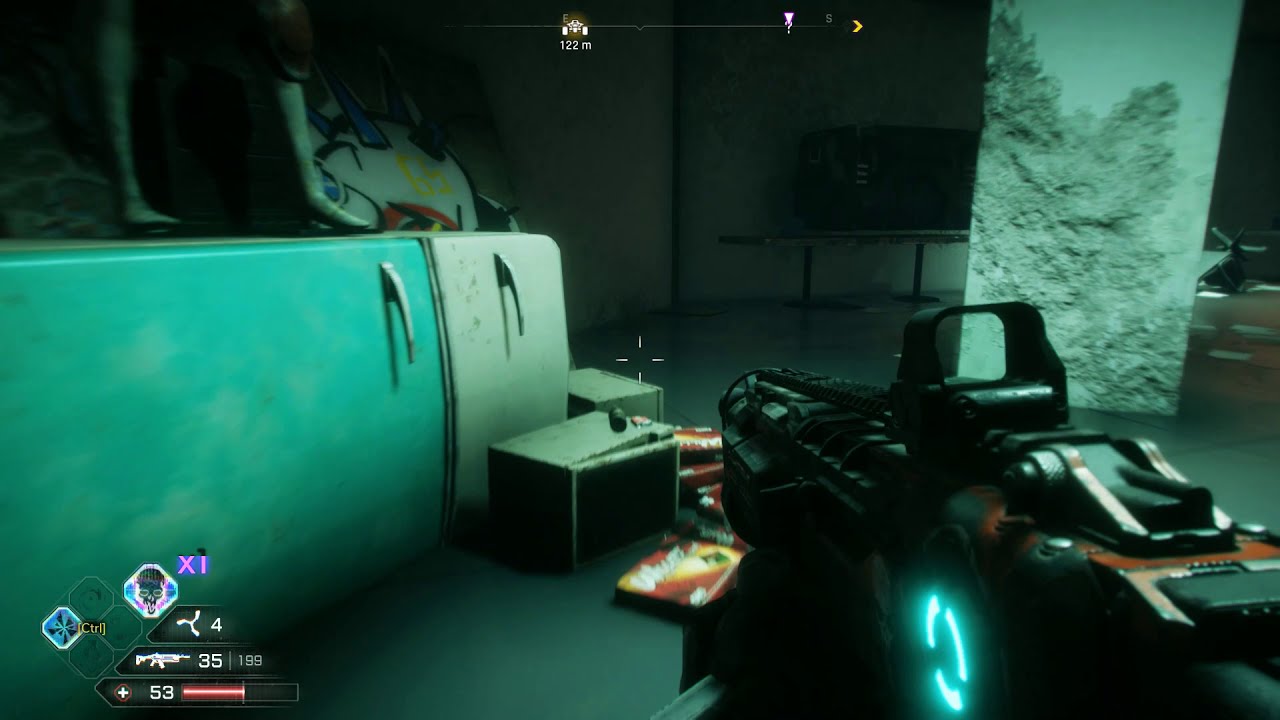The image is a screen grab from a first-person shooter video game, depicting a player holding a large, futuristic black gun with a blue circular design on its side, taking up the bottom right-hand corner of the screen. The gun's detailed features include a large barrel and sight, emphasizing its mechanical and imposing nature. At the bottom of the screen, various game stats such as a health bar, marked with the number 53 in white, and other status indicators are visible.

The game setting appears to be an abandoned building characterized by its dark, dilapidated environment. The concrete walls are adorned with graffiti, enhancing the sense of neglect, and the debris is scattered around the space. Prominently, an old-fashioned refrigerator, turquoise and white, lies on its side in the left part of the screen. Atop the refrigerator, bare feet are visible, suggesting someone is standing there, possibly an in-game character or adversary. In the background, behind the refrigerator, a vague advertising sign can be seen, adding to the eerie, post-apocalyptic atmosphere. The scene is devoid of any in-game text, allowing the disturbing ambiance and the detailed graphics to stand out.